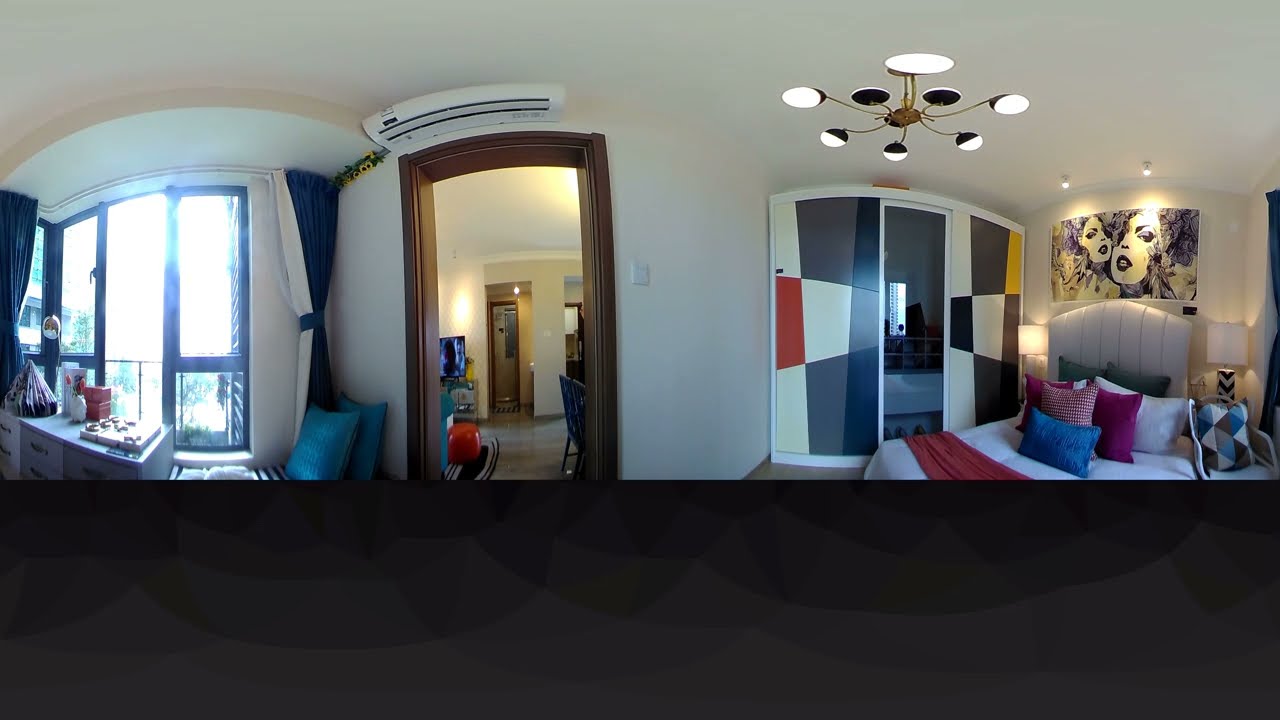This indoor image, seemingly an apartment, showcases multiple rooms beyond three doorways, all from a perspective that appears to be slightly distorted, possibly a 360 panoramic view. The predominant colors include yellow, blue, red, white and shades of black and brown. There’s a living room, a bedroom, and a bathroom visible. 

In the top left, there’s a sink with a mirror above it and a ceiling light fixture. The walls are yellow and the ceiling is pale yellow with round small light fixtures visible on the left-hand side. A striking blue, red, and white chandelier hangs prominently in the middle room. 

The bedroom, positioned centrally, features a small bed with a checkerboard green cover, a blue chair near a window, a red bag on the wall, white walls, wooden flooring, and a black window with wooden columns. There’s also a yellow wardrobe and a yellow, blue, and red chandelier-like light fixture with a candlelight appearance. To the right of the bedroom doorway is a bathroom with a shower stall. 

To the left, we see what appears to be a living room with blue chairs, one red chair, a dining room table, and a painting of two people on the wall. The setting seems to capture daylight filtering through, giving an impression that the photo was taken during the middle of the day.